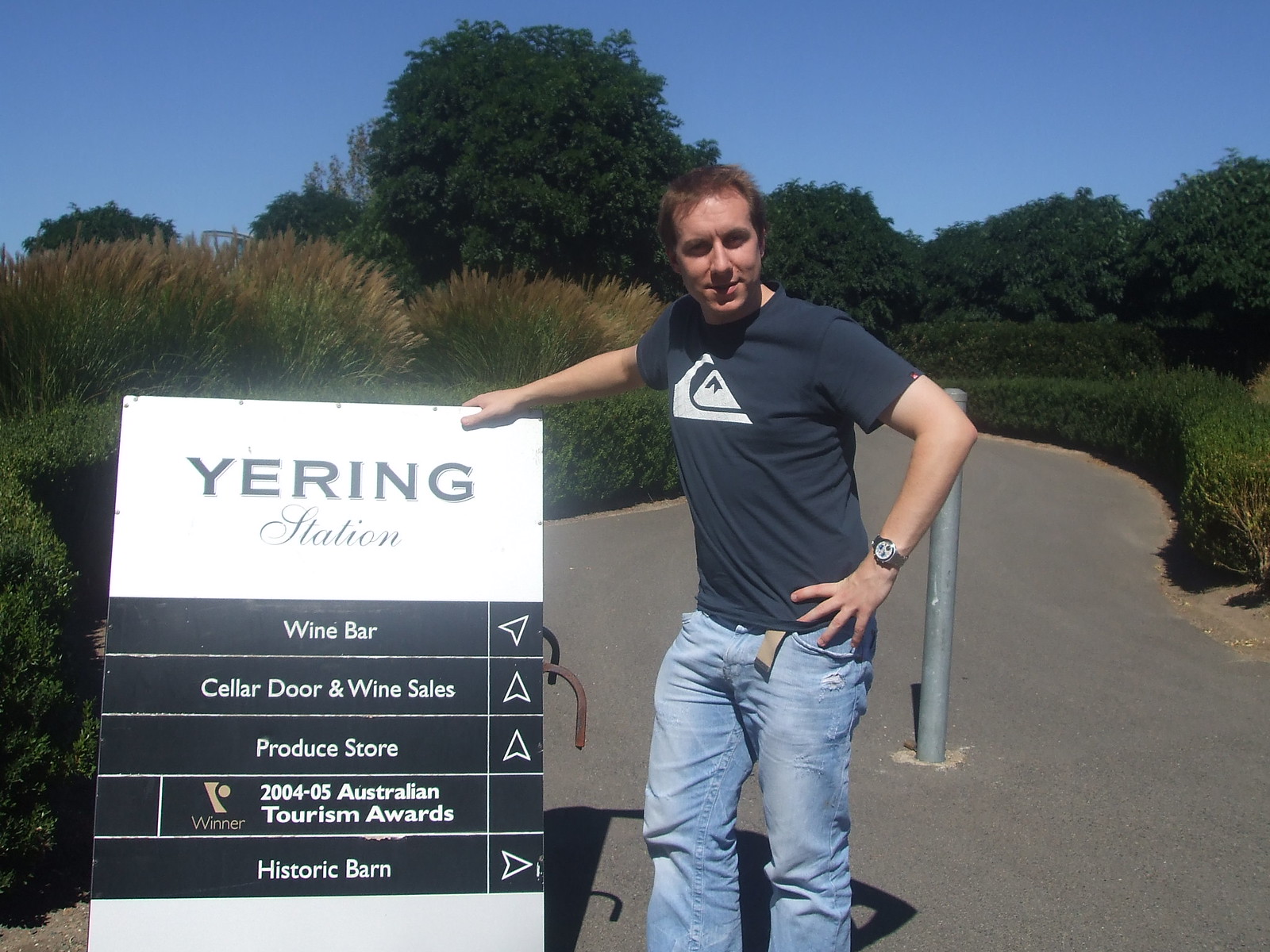In this photorealistic image, a young Caucasian man with brown hair stands casually on a grey path that stretches into the distance, surrounded by lush green trees and bushes. He's wearing a navy shirt with a light white mountain icon on the chest, blue jeans, and a beige belt, along with a watch on his left wrist. He rests his right hand on his hip while his left hand is extended, resting on a sign beside him. The white sign reads “YERING STATION” at the top in black, boxy capital letters. Below this, "Station" is written in black cursive. The sign also features a black section indicating directions: "Wine Bar" with an arrow pointing to the left, "Cellar Door and Wine Sales" and "Produce Store" both with arrows pointing up, "2004-2005 Australian Tourism Awards," and "Historic Barn" with an arrow pointing to the right. A bright blue sky can be seen in the background, adding to the serene atmosphere.